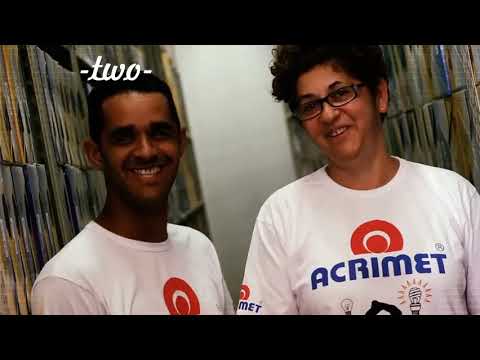The image features a small, horizontal, rectangular photograph with thick black borders at the top and bottom. It depicts two smiling individuals, likely of Hispanic descent, standing in what appears to be a file storage area filled with shelves of paper files. The person on the left is a man with short black hair, wearing a white t-shirt with a distinctive red logo resembling a target but flat on the bottom. Above his head, in cursive, the word "two" is written in lowercase. The woman on the right has short, curly brown hair and wears black glasses. She is also wearing the same white t-shirt, which reads "Acrimet" in big blue letters across the center, along with the same red target-like logo. Below the "Acrimet" text on her shirt are illustrations of two light bulbs: one traditional bulb without any triangles around it, and a high-efficiency bulb with small yellow triangles indicating it is lit.